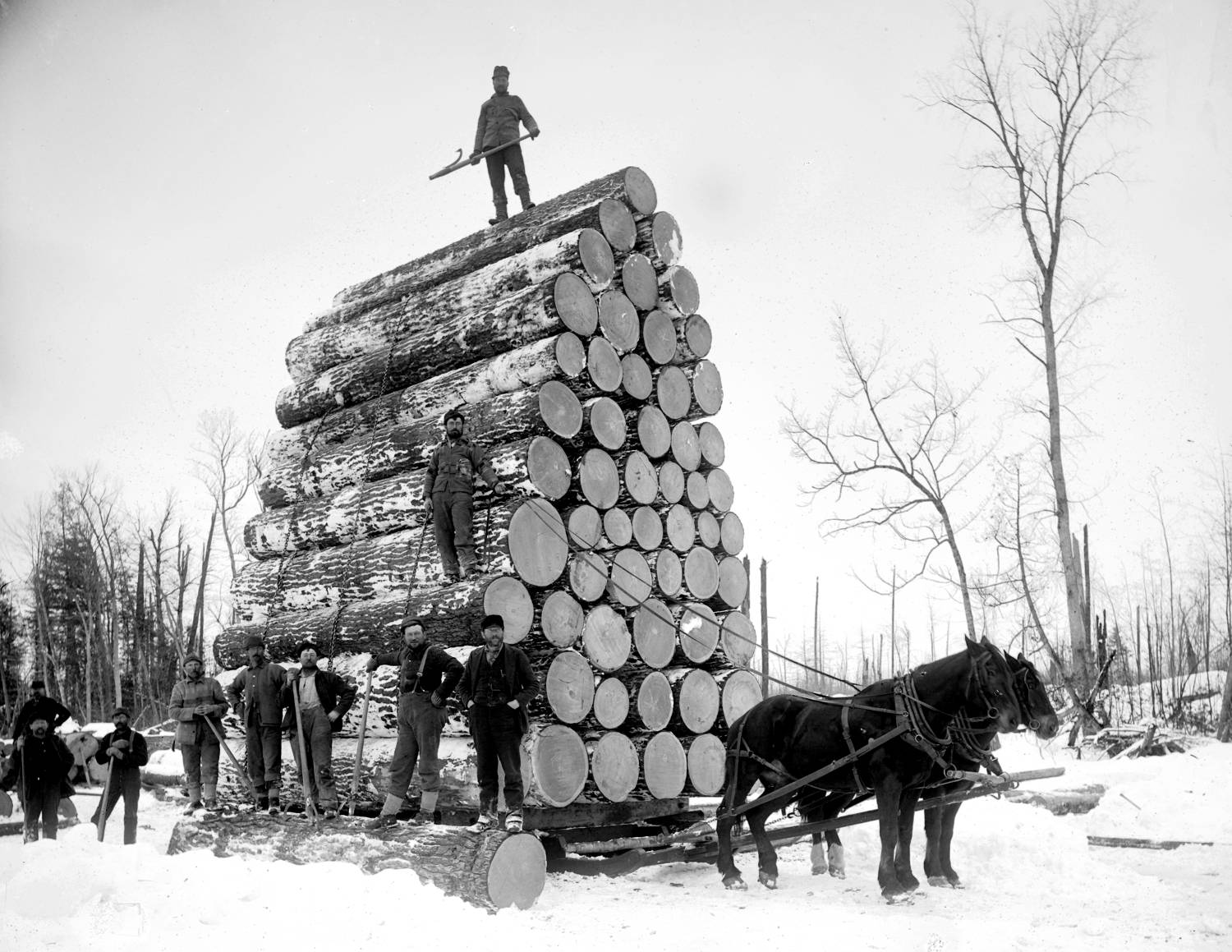This is a large, old black-and-white photograph taken outdoors during the daytime in winter. The image presents a striking scene of industrious labor amidst a snowy landscape with barren trees and a few scattered pine trees to the left. Central to the composition is an enormous pyramid-shaped pile of evenly cut logs, dusted with snow, with a man standing at its pinnacle holding a pole or hook. Another man is midway up the structure, on the third level of logs. 

On the ground level, five men are standing on a log, holding shovels or axes, hands on hips, posing for the camera, with a couple of other men to the left, standing on the snow. Prominently featured are two dark horses, yoked and facing right, appearing to be harnessed to a sled loaded with these massive logs. A man standing on the ground holds their reins, adding a dynamic element to the scene as if they're poised to pull the hefty load. The sky appears light gray, adding to the nostalgic aura of this compelling, well-composed photograph.